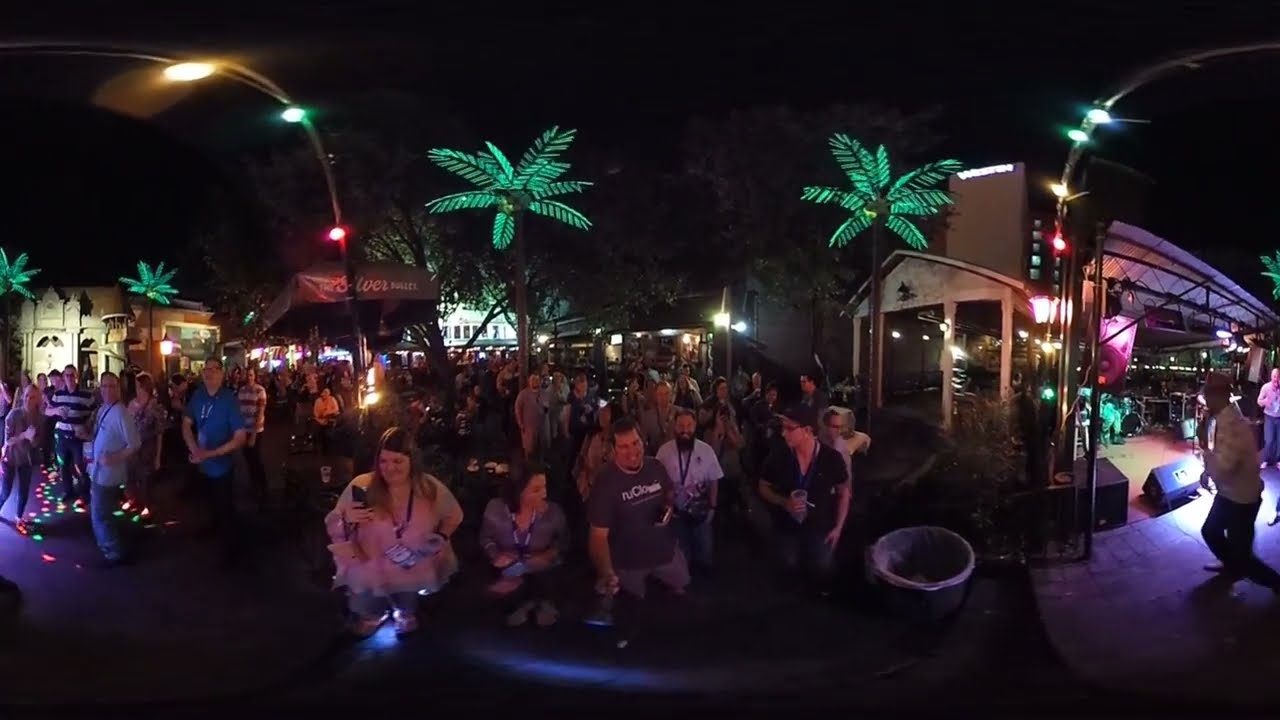The image captures a bustling outdoor club or bar during a tropical-themed party, possibly set in Florida. The scene is centered around a large crowd of hundreds, if not over a thousand people, who are dancing and mingling. In the middle of the image, people are gathered around a black console-like table, which appears to be a DJ setup where attendees can either create or listen to music, adding to the energetic atmosphere. To the right of the image, a four-member band is playing vibrant tunes under a canvas roof with metal framing, illuminated in blue light. This stage area is further accentuated by four artificial palm trees adorned with green lights where their leaves would be, contributing to the tropical vibe. On the left, there’s another stage, partially visible, with alternating green and red floor lights, indicating possibly another performance space or show. Surrounding the scene are casual stores and buildings, enhancing the feel of a lively marketplace or plaza, buzzing with nightlife and festivity.